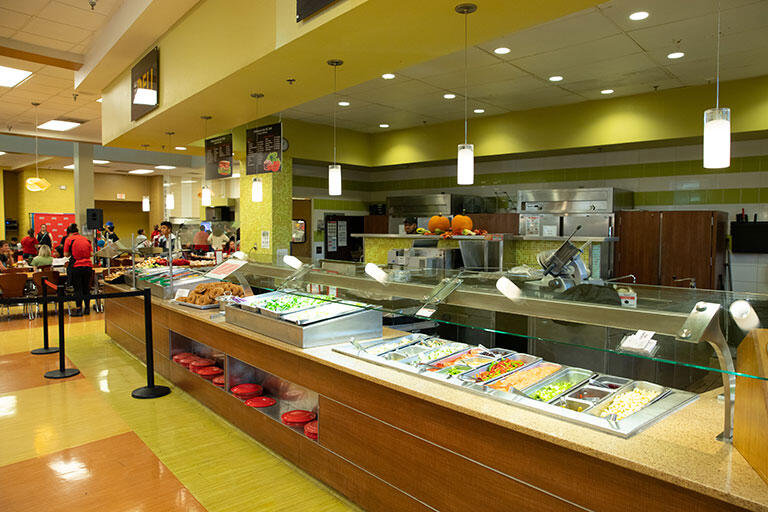The image captures an expansive cafeteria or buffet-style setting with a distinctive yellow-green hue to the walls and a mix of white ceiling tiles outfitted with both square fluorescent and pendant lighting. Central to the image is a long, self-serve food bar adorned with a clear glass sneeze guard, built into a yellowish-tan stone or quartz countertop with a wood-finished base. The buffet features various food items, including trays of donuts or bagels and what appears to be a salad bar, possibly alongside other sections like a taco bar and additional sides. The floor sports a vibrant mix of light green, yellow, and orange tiles. Towards the back of the image, there is a seating area filled with tables and chairs, where several people are sitting. The entire room glows with a warm, yellow light, enhanced by multiple hanging pendant lights that dot the ceiling.